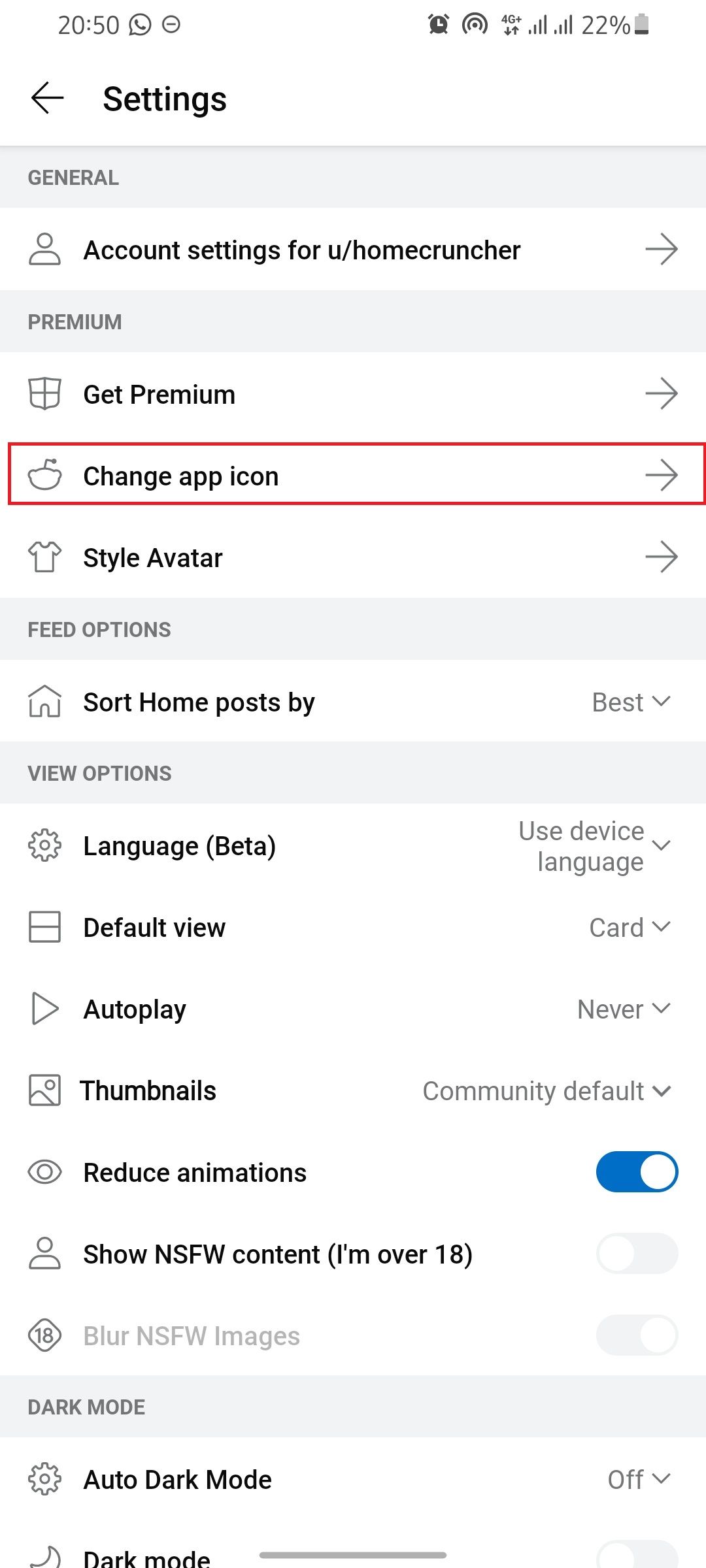This detailed caption provides an in-depth description of the phone screenshot, highlighting the various sections and settings available:

---

This screenshot depicts the settings menu of an Android phone application. The settings are categorized into several sections including General, Premium, Feed Options, View Options, and Dark Mode.

In the General section, the account settings are specified with the username "you/home cruncher". The Premium section offers options to "Get Premium" and "Change App Icon", with the latter highlighted by a red outlined rectangle. Also listed here is "Style Avatar".

The Feed Options section allows the user to sort home posts, with "Best" currently selected. This option features a drop-down menu icon next to it, suggesting more sorting preferences are available.

The View Options section includes a variety of settings:
- Language
- Beta
- Default View
- Autoplay
- Thumbnails
- Reduce Animations (this option is toggled on)
- Show NSFW Content (indicated with "I'm over 18" in parentheses)

A grayed-out setting "Blur NSFW Images" appears under this section, indicating it is currently unavailable or disabled.

Finally, the Dark Mode section offers two settings: "Auto Dark Mode" and "Dark Mode".

This detailed view of the settings menu offers a comprehensive look at the customization options available within the app.